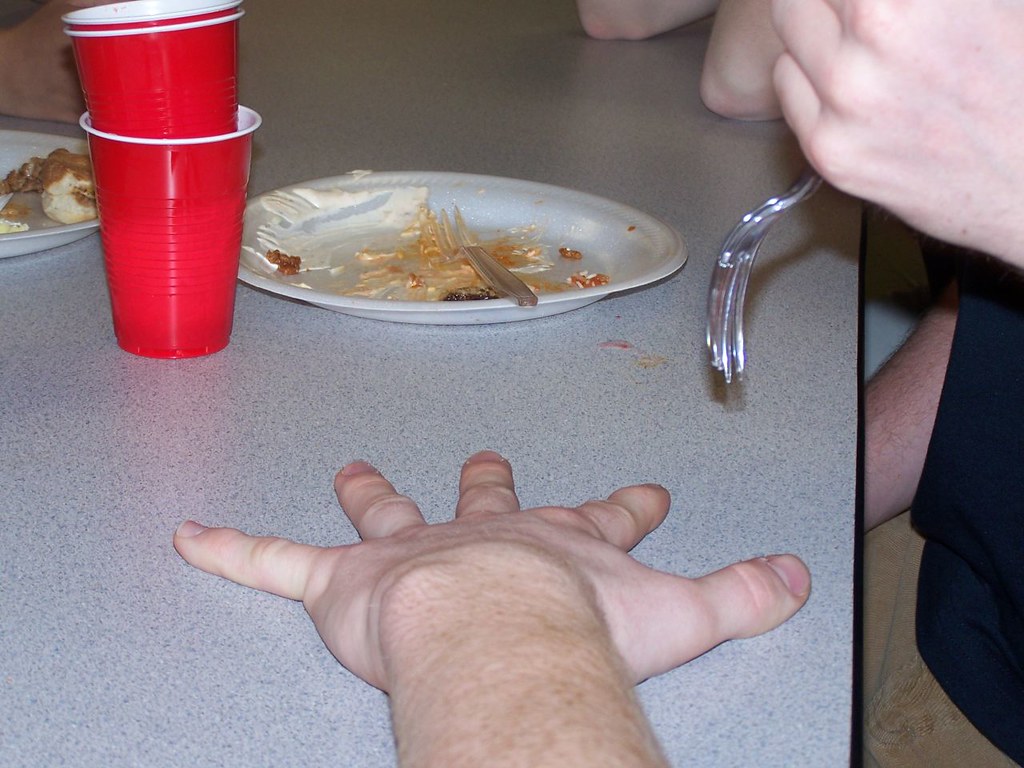In the photograph, a person's hand is prominently featured, laid out flat with fingers splayed in a star pattern on a grey dining table. Nearby, a paper plate with food remnants and a plastic fork sits. To the left of the hand, three red Solo cups are stacked. In the background, another plate with some food can be seen. Positioned to the right, partially visible, is another individual, identifiable by their black clothing. This person holds a clear plastic fork in their left hand, seemingly preparing to bring it down towards the outstretched hand. Additional details include the visibility of elbows resting on the table at the far ends of the image, indicating other people around the table. The scene suggests the start of a playful game involving the fork and the spread-out fingers.